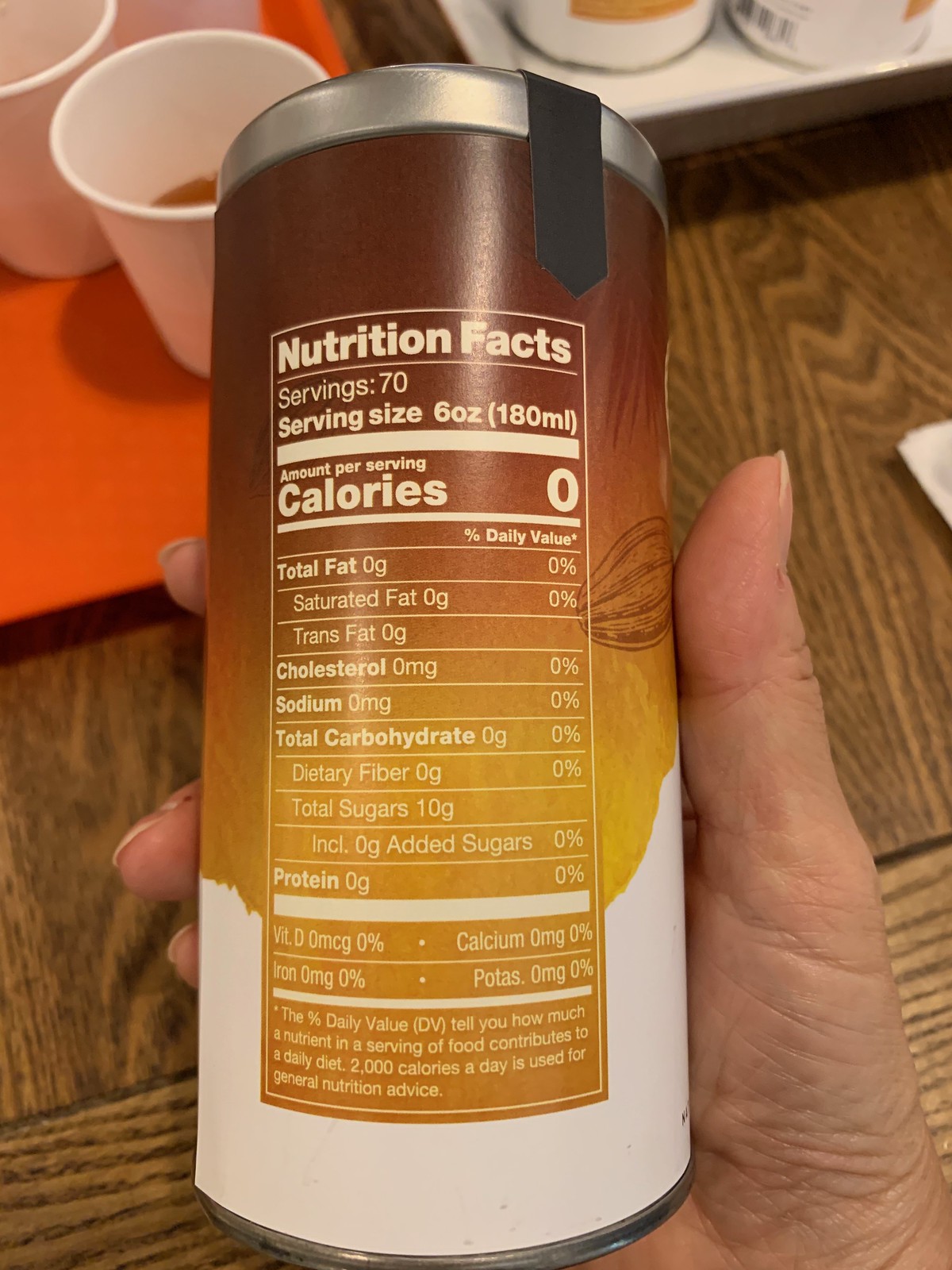The color photograph features a close-up of a person's right hand holding a cylindrical metal can, likely aluminum, with a silver cap secured by a piece of black tape. The can's design is predominantly brown with a white section at the bottom. The person is inspecting the Nutrition Facts label, which reveals detailed information: the container holds 70 servings, each serving size is 6 ounces or 180 milliliters. The nutritional values per serving are: 0 calories, 0 grams of total fat, saturated fat, and trans fat, 0 milligrams of cholesterol, 0 milligrams of sodium, 0 grams of total carbohydrates, dietary fiber, and added sugars, but 10 grams of total sugars. Additionally, vitamins and minerals such as Vitamin D, calcium, iron, and potassium are all listed at 0% daily value. The label includes a note explaining that the percent daily value (DV) is based on a 2,000-calorie diet. In the background, there is a wooden table where the person's hand rests, visible along with an orange tray positioned in the upper left corner and two white disposable cups, likely containing a drink, partially filled with a brown liquid.